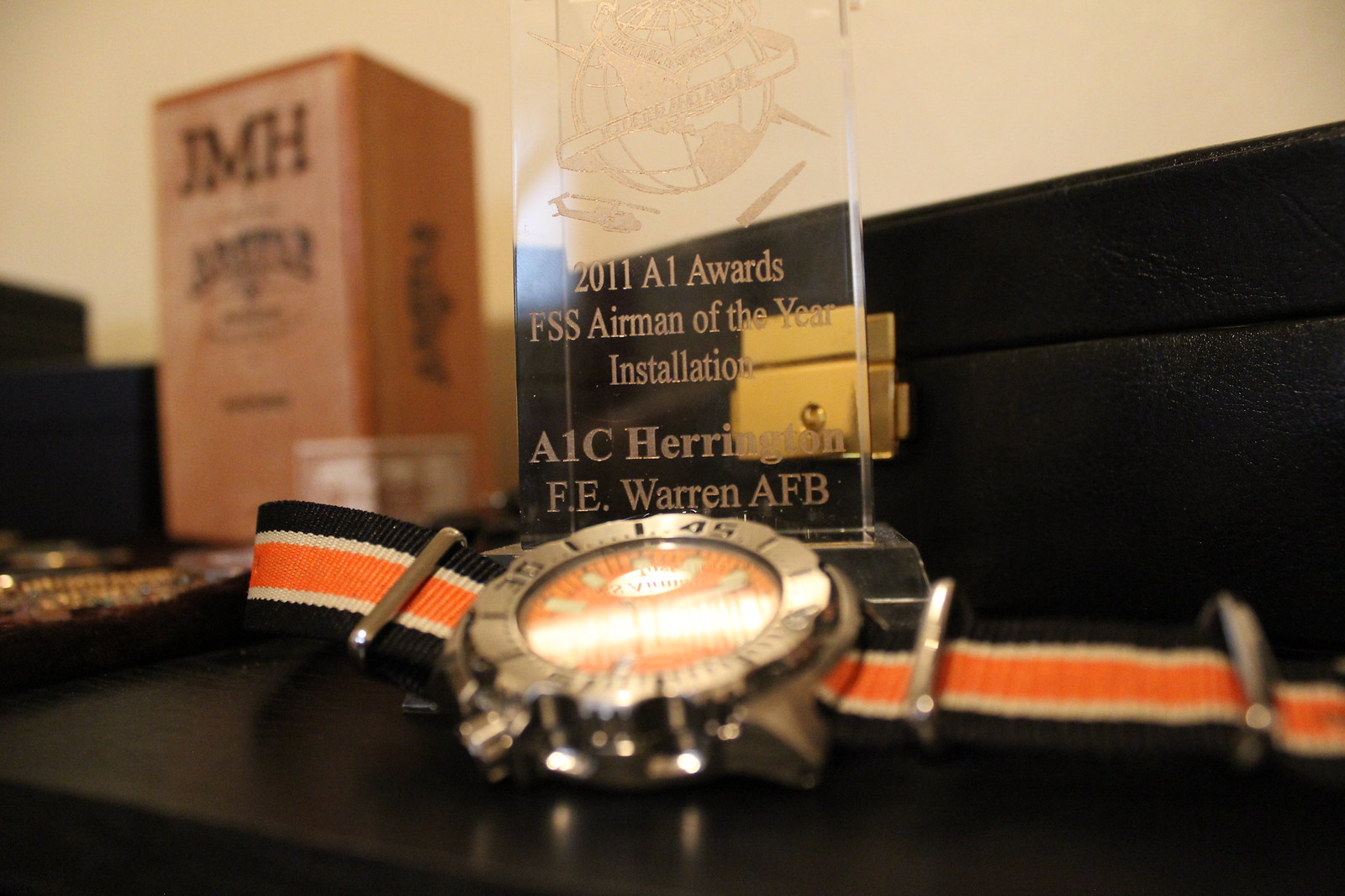This close-up image highlights a glass award and a watch resting on a black leather surface, with a tan-colored wall in the background. The main focus is a clear, vertically rectangular glass award with an etched design at the top, possibly depicting a globe. The inscription on the award reads: "2011 A1 Awards FSS Airman of the Year Installation, A1C Harrington, FE Warren Air Force Base." Flanking the award on the left is a blurry orange-colored wooden box embossed with black letters "JMH" and other indistinct designs. In front of the award lies a distinctive watch with an orange face and a silver outer ring. The watch features a fabric band with alternating blue, orange, and white stripes, and metallic buttons and numerals marked at various degrees around the edge. The scene is set on a black leather object with a subtle backdrop, showcasing an elegant display of accomplishment and timepiece.